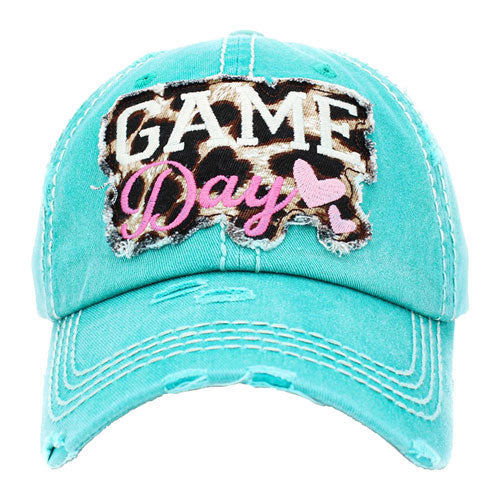This photograph showcases a front view of a well-worn, teal denim baseball cap. The cap exhibits purposeful distressing along the edges of the bill and other parts of the fabric, giving it a tattered appearance. Contrasting white stitching enhances its design, with three rows visible around the bill. The focal point of the cap is a prominently sewn patch on the front, which reads "GAME DAY." The word "GAME" is in bold white letters, while "DAY" is in pink cursive script. Adding to the charm are two light pink embroidered hearts next to "DAY". This text and the hearts are set against a distinctive leopard or cow print background, featuring brown and white spots. The overall effect is a vibrant yet rugged cap with intricate details, set against a plain white backdrop.